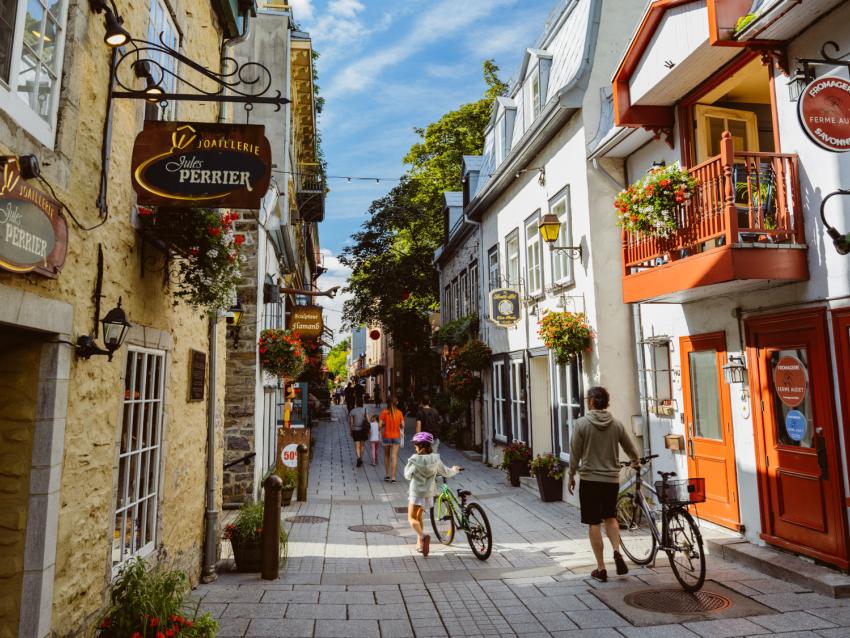This image, with near-square horizontal alignment, captures a charming village alleyway between older buildings. On the left, the alley is bordered by a series of two to three-story buildings made of brown stone, with one prominently featuring a sign that reads "Jules Perrier." Across from this, on the right, stands a white stone building with dark wood elements, including a ground-level door and a balcony adorned with hanging flowers and open doors.

The alley itself is relatively wide, paved with light gray stones, and bathed in sunlight under a blue sky with feathery white clouds. Walking down the pathway are various people: a man to the right pushing an older style bike, and a child with a purple helmet walking their bike. Further down, other pedestrians can be seen, including someone in an orange shirt, a child in a white shirt, and a woman with a purse wearing a gray shirt.

In the background, additional buildings and some greenery contribute to the cozy, picturesque ambiance of this scene, giving the impression of a peaceful, leisurely day in a quaint village setting.